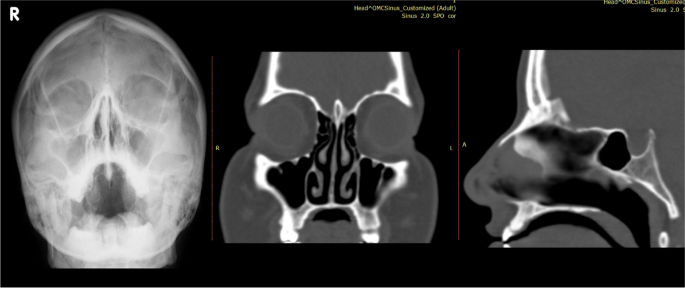The image presents three X-ray scans against a black background, each displaying different views of the head and neck region. The leftmost scan clearly shows a frontal view of a person's head, highlighting the nose, eye area, and open mouth, depicted in white and gray tones. The middle scan is ambiguous but features a notable black central area surrounded by white lines and extensive gray shading. The rightmost scan offers a side profile of the head, detailing the forehead, eye socket, nose, and sinus region, again utilizing a combination of white, gray, and black shades. The scans are accompanied by a white letter "R" in the top left corner, with additional text in yellow positioned at the top middle and top right corners of the image.